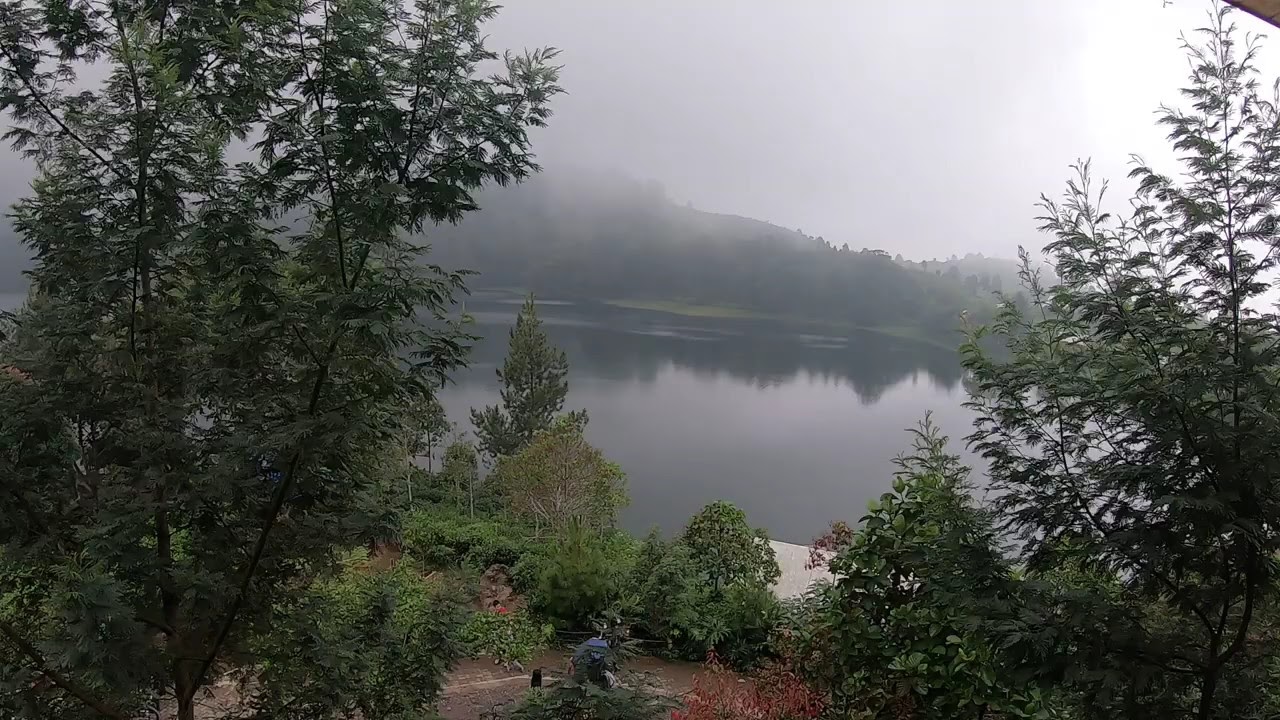The image depicts a serene, foggy lake scene, possibly captured in the early morning. Overlooking the lake from a hilltop, the view is slightly obscured by a dense fog and an overcast sky, casting a soft, muted light over the landscape. The foreground is framed by many trees on the left and right, some of which seem to extend into the lake or overlook it. A worn dirt path or dock juts out slightly onto the lake's edge. The still water reflects the distant hills and additional trees from the opposite side, enhancing the depth and tranquility of the scenery. Although slightly faded in the mist, hints of a structure and a person in a red shirt can be discerned near the shore. The natural palette of greens and browns blends harmoniously with the dark blue hues of the clear, unpolluted lake, evoking a calm, reflective atmosphere typical of a Midwestern landscape.